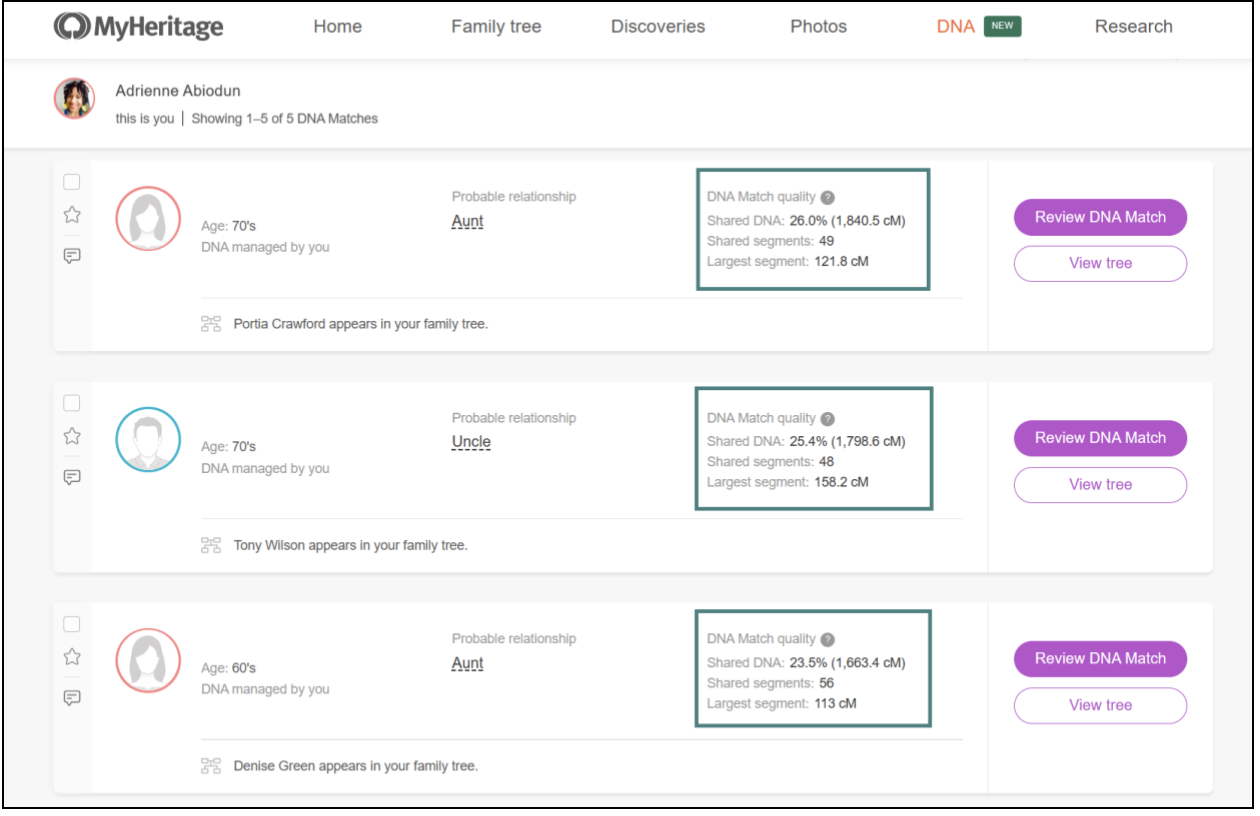This is a screenshot of a MyHeritage webpage displaying detailed DNA match information. At the top, a white navigation banner presents options such as "Home," "Family Tree," "Discoveries," "Photos," and "DNA," with the "DNA" section marked as new and under research. 

Prominently featured is Adrian Abaddon, who is conducting this research and has identified five DNA matches. The first match, whose age is in the 70s, has their DNA managed by the user. Portia Crawford, identified as a probable aunt, appears in the user's family tree. The match details include DNA match quality, shared DNA, shared segments, and the largest segment.

The second match, also in their 70s, is indicated as an uncle named Tony Wilson, who also appears in the family tree. This match reports a DNA match quality indicating 25.4% shared DNA, distributed over 48 segments, with the largest segment being 56.

The final match shown, an aunt in her 60s, has a DNA match quality displaying 23.5% shared DNA over 56 segments, with the largest segment being 113. The webpage provides a way to explore potential ancestry connections through these DNA match details.